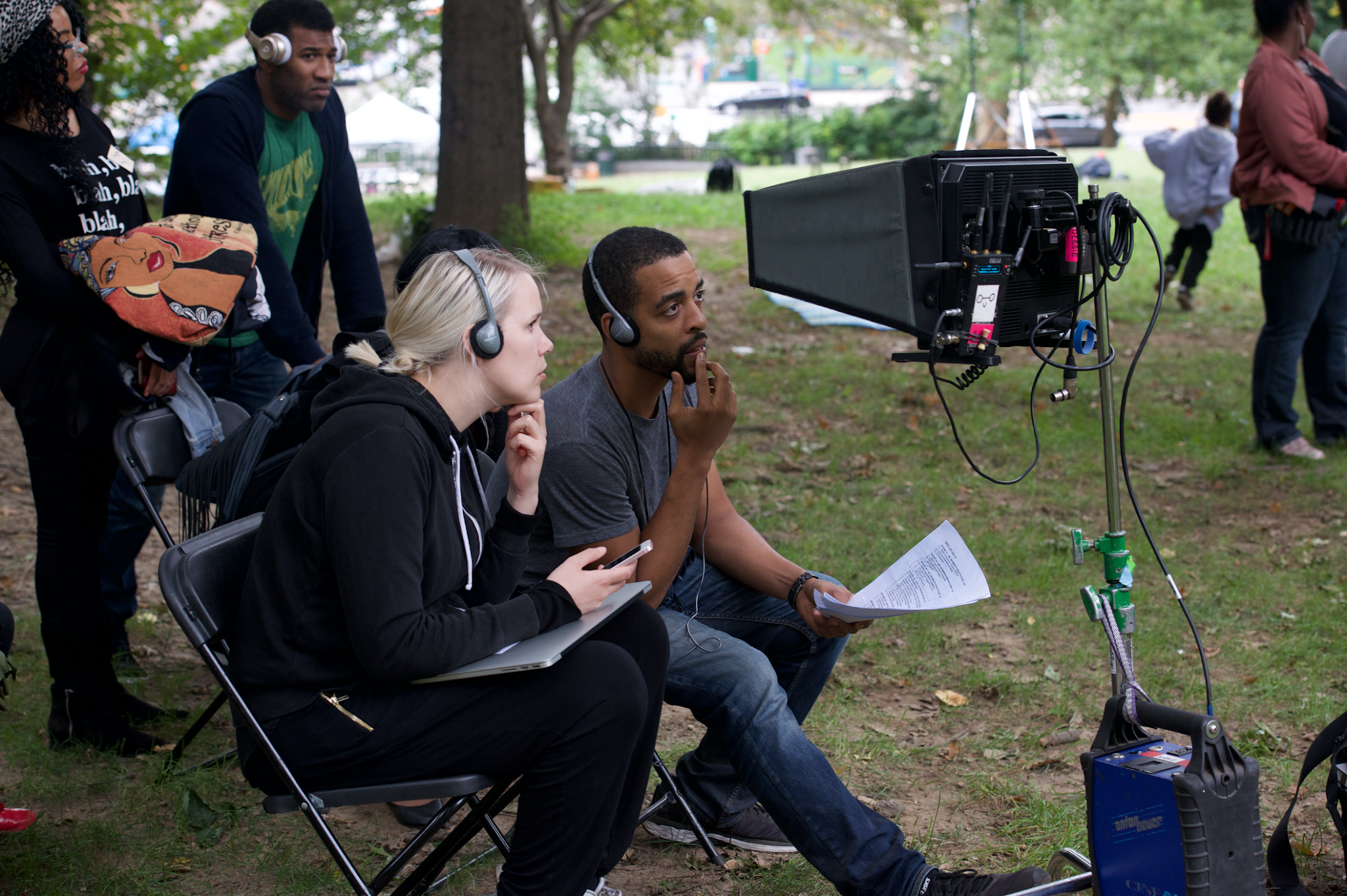The color photograph depicts the bustling atmosphere of a movie set situated in a public park, captured in a landscape orientation. In the foreground, two individuals are seated in folding chairs, both wearing headphones and focused intently on a piece of camera equipment placed on the grass. The equipment, which has a gray cover to mitigate monitor glare, displays either a live feed or a replay of the scene being filmed. 

The person on the left, identified as independent script supervisor Tamara Henson, has blonde hair and a folded laptop on her lap. Next to her is an African-American actor, Rashid Green, holding a script in his hand. Both figures are dressed casually in t-shirts, sweatshirts, and jeans, reflecting the informal yet concentrated atmosphere of the set. 

Standing behind them are two more crew members: a woman holding a bag and sporting a sweatshirt with unreadable white text, and a gentleman with headphones resting on his forehead. The background reveals a serene park scene with trees and distant cars, along with a small group of onlookers and additional crew members scattered around, some wearing headphones. A few kids can be seen playing, adding to the public park setting. The photograph captures a slice of filmmaking amidst everyday park life, blending the technical and the casual with a touch of realism.